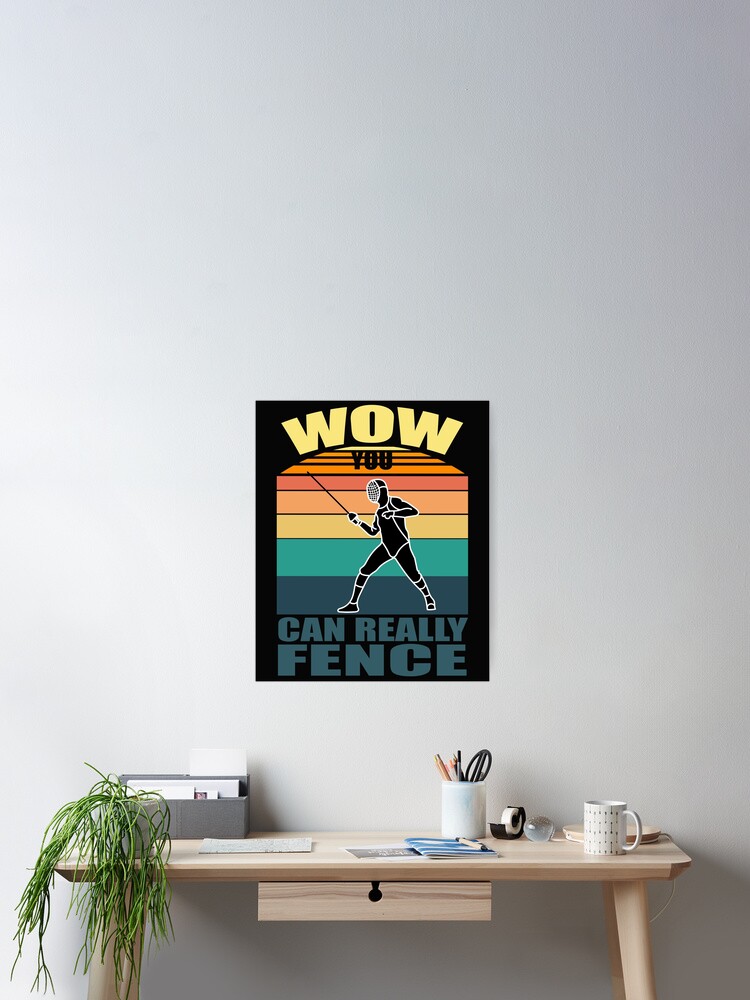This is a picture of a small rectangular wooden desk with a light brown finish and a front drawer featuring a black knob. The drawer has a keyhole at the top, though it doesn't seem functional. On the right side of the desk is a small white desk lamp, alongside a white coffee mug. Next to the mug sits a black tape dispenser with tape in it, and a white or glass container holding pencils, pens, and possibly scissors. In the middle of the desk, there are some scattered papers and a blue booklet. A gray organizer box, presumably filled with papers, is positioned toward the back left corner of the desk. A small green potted plant with drooping stick-like leaves is also on the left side. 

Above the desk, attached to the white wall, is a black poster with a rainbow design in the background. At the top of the poster, the word "Wow" is written in yellow, followed by the phrase "you can really fence" in dark teal. The poster features an image of a fencer in full gear.